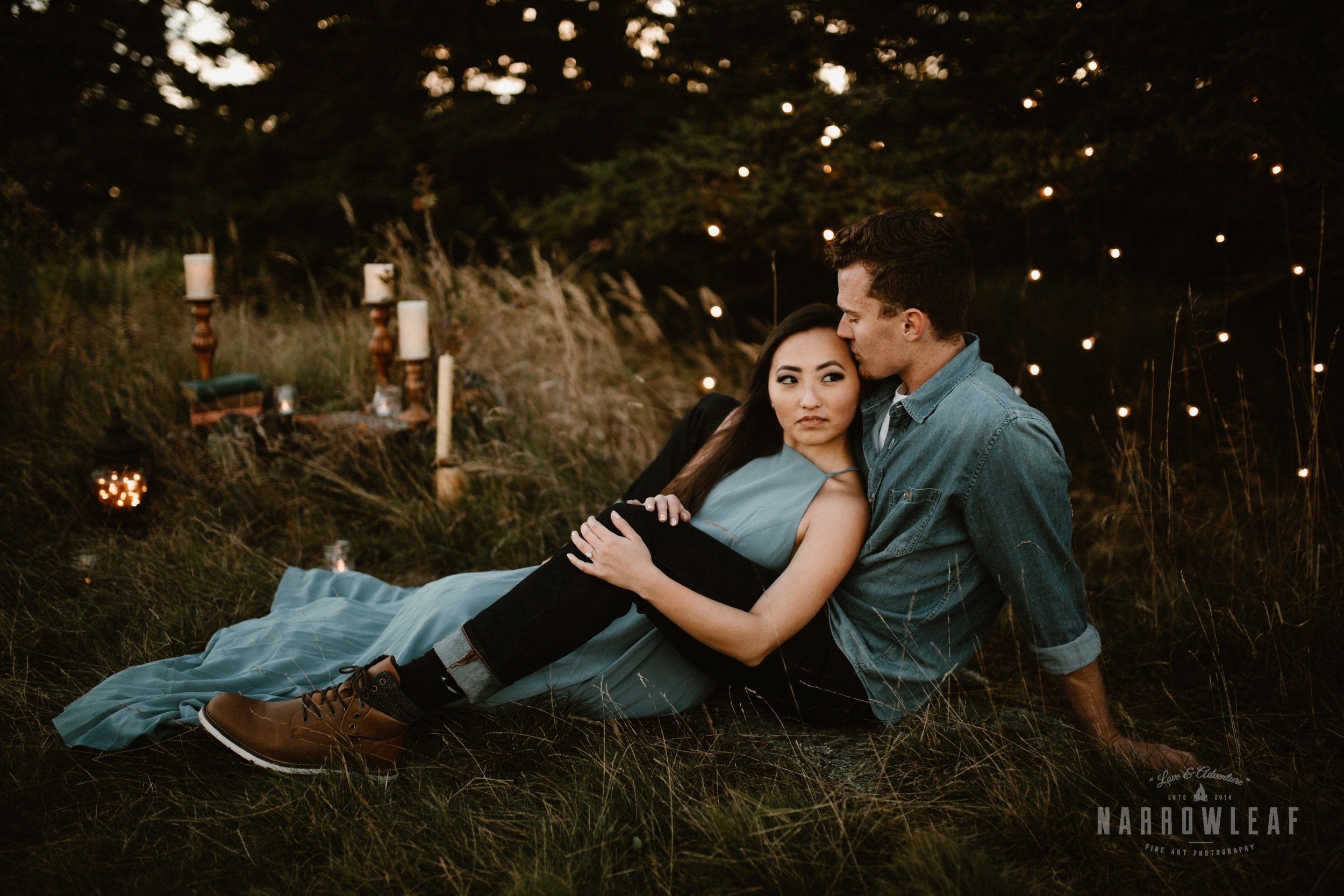This captivating outdoor advertising image, styled photographically, captures an intimate moment between a couple lying on the grass at dusk. In the foreground, a Caucasian man with short brown hair sits up, dressed in a light denim blue, long-sleeved button-up shirt, dark blue (or black) pants, and brown shoes. He tenderly bends down to kiss the forehead of an Asian woman with long black hair, who is elegantly reclined against his chest. She wears a long, sleeveless light blue dress and holds onto his leg.

The setting features a grassy field interspersed with tall green and tan, wheat-like grasses. Scattered ambient lights glimmer like fireflies around the couple, contributing to the romantic atmosphere. In the top right-hand corner, a cluster of three to four unlit white candles on wooden candlestick holders sits near some trees, adding to the rustic charm. A small fire flickers on the left edge of the image, while the background reveals a serene yellow-orange sky blending with the silhouettes of trees.

In the bottom right-hand corner of the poster, a logo and text appear, with the most legible words being "narrow leaf." The overall composition, enhanced by these subtle details, conveys a blend of love and adventure, inviting viewers into the serene, heartfelt moment shared by the couple.